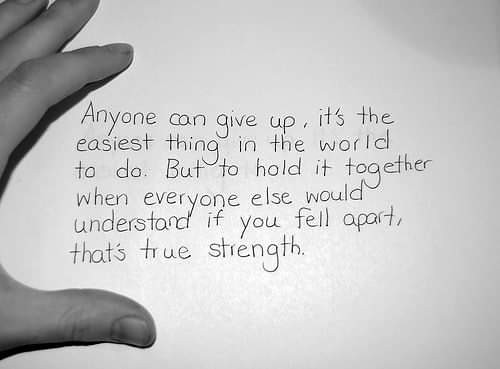In this black and white image, a Caucasian hand is resting on a white piece of paper, securing it in place but not grasping it firmly. The hand, positioned on the left side of the paper, has the thumb horizontal to the bottom of the frame, with the index, middle, and ring fingers pointing slightly upward. The pinky finger is not visible. The paper is centered in the frame and features a handwritten message in black text that reads, "Anyone can give up. It's the easiest thing in the world to do. But to hold it together when everyone else would understand if you fell apart, that's true strength." The background is a plain white, with some shadow in the top right corner, suggesting an unseen round object casting it. Despite some JPEG artifacting around the letters, the text remains quite legible, hinting that this might be an older photo that has been compressed.